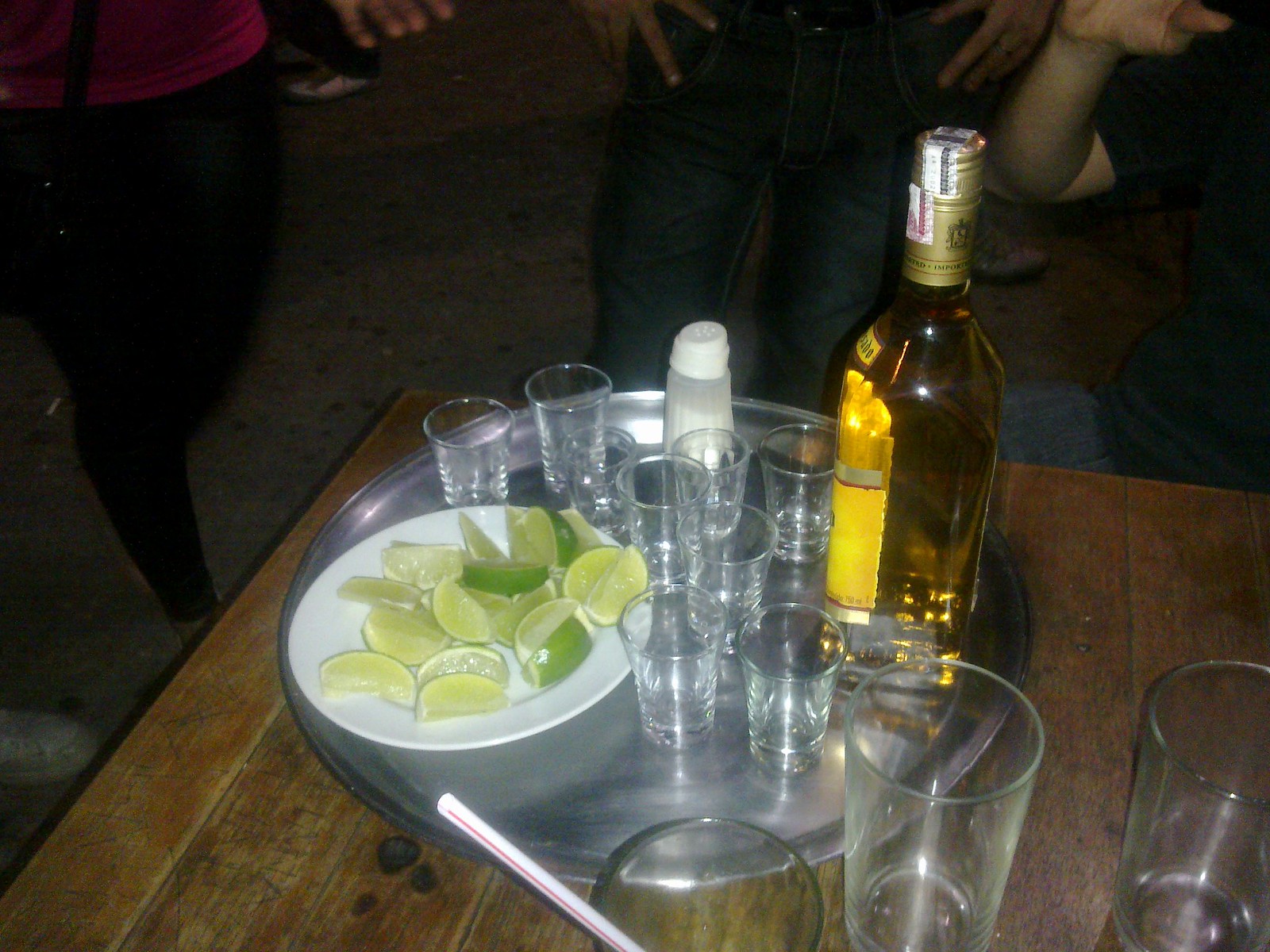This photograph taken at a party features a round silver platter centrally placed on a slightly faded wooden table. The platter holds a variety of items, including a bunch of empty, translucent shot glasses, a white dessert plate with lime wedges displaying their yellowish-green interiors and vibrant green peels, and a small salt shaker with a white cap containing a white powdery substance. Dominating the right side of the tray is an unopened bottle of brown, translucent tequila with a gold label and a cork that has a goldish hue and black text.

Surrounding the platter on the table are additional items: two tall empty glasses, one with a straw marked by a red stripe. The background reveals a gray, dirty floor and the lower bodies of at least five individuals, suggesting a lively social setting. Visible among these people are a woman in black pants with a red shirt, a man in dark blue jeans, and another person of indeterminate gender wearing a black shirt. Some of the individuals have light complexions while others have darker complexions, and one person is carrying a purse. The scene captures a dynamic party atmosphere with elements of social interaction and festive preparations.